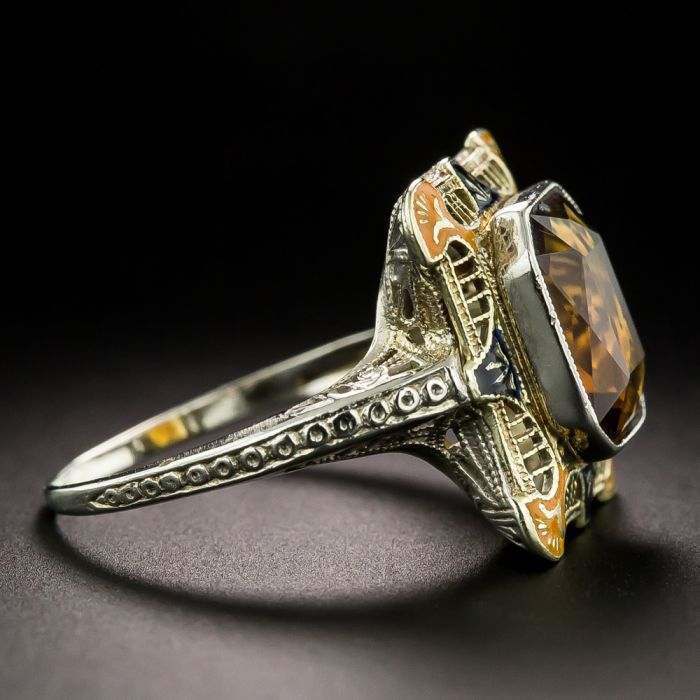This is an extremely detailed close-up photograph of an ornately designed ring. The ring features a band crafted from either silver or white gold, adorned with a series of etched circles that extend most of the way down the band, stopping near the bottom. The band flares out towards the ring’s setting, which houses a striking rectangular amber gemstone. This gemstone, a deep tea-colored amber, is beautifully cut and has a lustrous shine. The gemstone is encased in a silver housing with intricate designs around its edges, featuring orange and black hues with delicate flower-like patterns. The background of the image is a stark black, which highlights the ring's details, and the ring itself is resting on a dark charcoal gray surface that reflects its shadow, adding depth and contrast to the photograph.